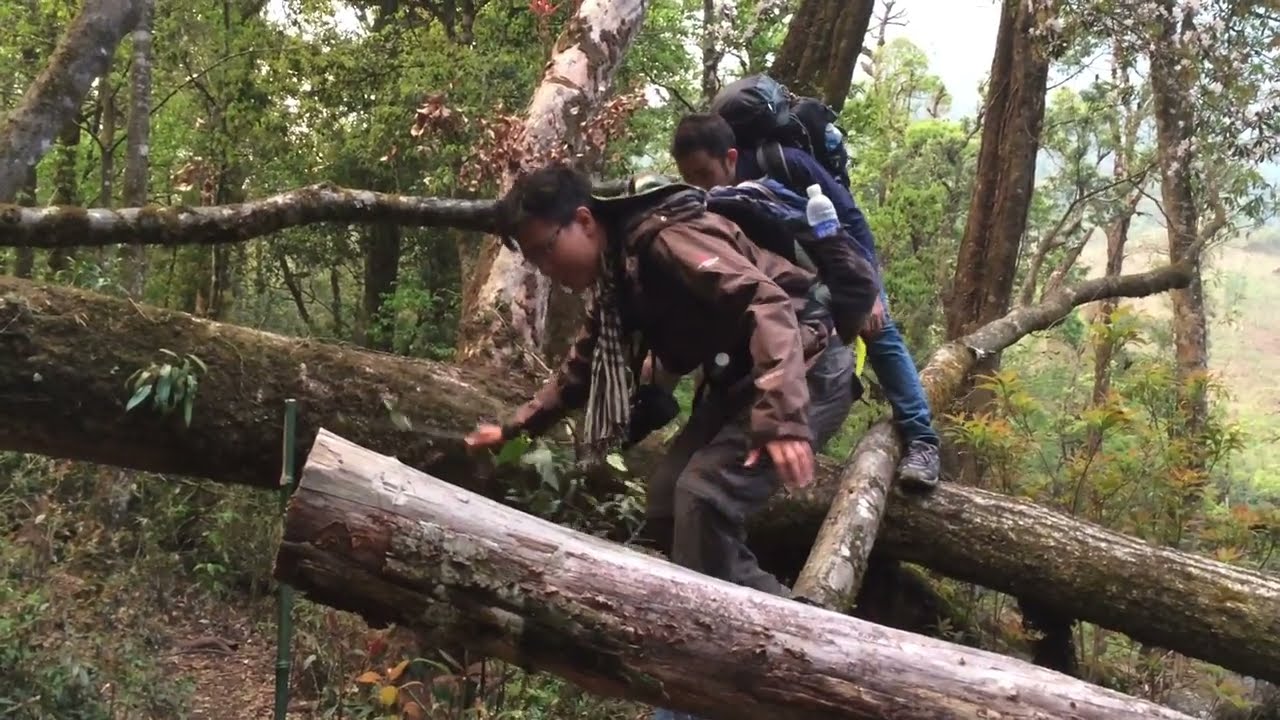In the center of this outdoor, forest scene, two men traverse a series of downed trees. The heavily wooded area features dirt, various tree trunks, and sparse patches of green foliage. The man on the left wears glasses, a brown jacket, a whitish scarf, and dark gray pants. He carries a backpack with a water bottle and steadies himself with his left hand splayed on a tree trunk, while his right hand hangs free at his side. The man on the right, standing on a log, is dressed in a dark blue long-sleeve shirt with blue jeans, hiking boots, and a black backpack. He also has a pouch across his chest. Both men are navigating the logs amidst the shaded forest floor with an overexposed sliver of sky visible in the upper right part of the image. Various colors, including green, brown, tan, gray, blue, and white, are present in the natural surroundings, highlighting the serene yet intricate setting of their hike.